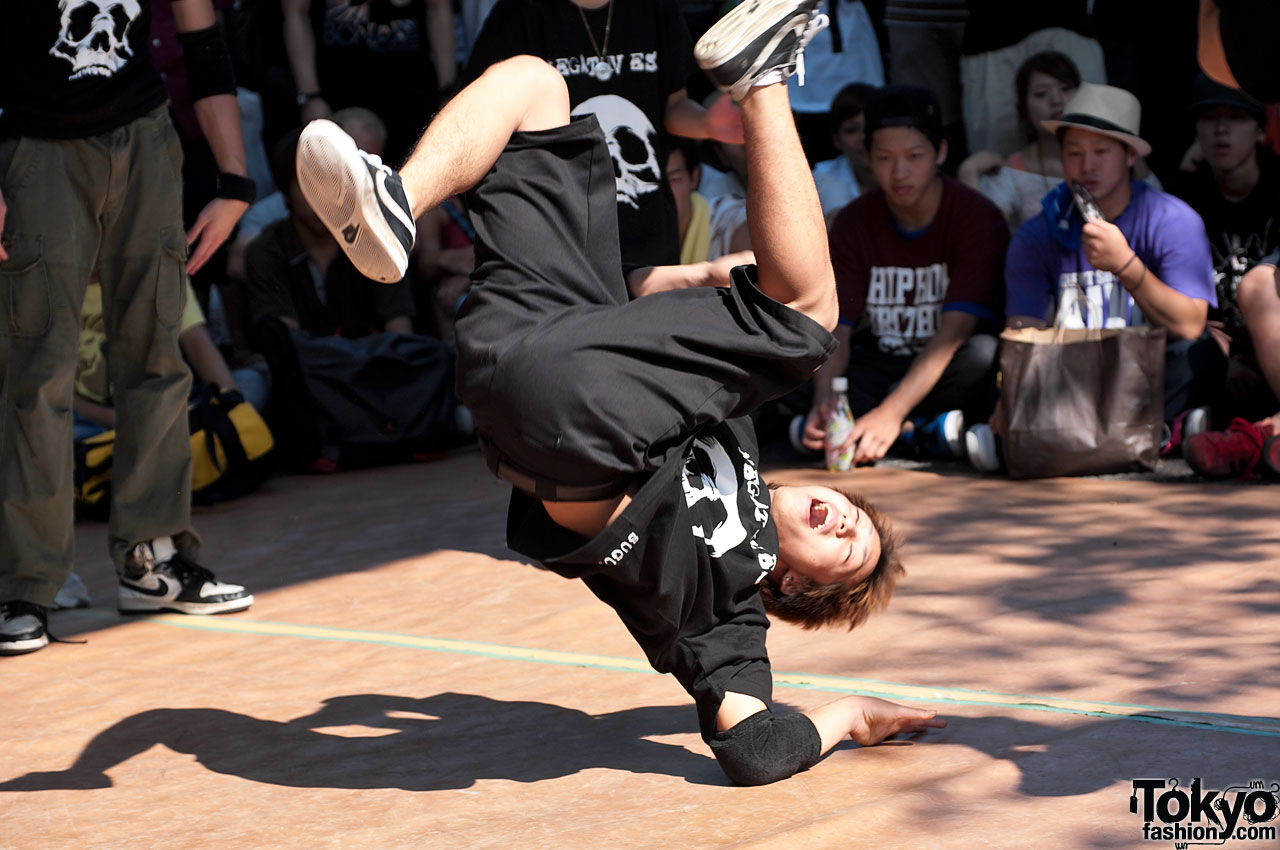In this captivating photograph taken in Tokyo, a dynamic young male breakdancer showcases his impressive skills. The lower right corner of the image displays a small logo reading "tokyofashion.com". The dancer, with his vibrant red hair and open mouth, is captured mid-move, expertly balanced on his left forearm which is bent at a 90-degree angle. Both his legs are suspended in the air, bent at perfect right angles, creating a striking visual. He is dressed entirely in black, including a black graphic t-shirt featuring a white skull design, black shorts, and black sneakers with white soles. Adding to the intense atmosphere are protective black elbow pads. Surrounding the performer, an audience comprising mainly of Asian individuals watches intently, with some dressed in matching graphic t-shirts. The scene is set on a reddish ground with a noticeable stripe running through the middle, further highlighted by the many shadows cast by the onlookers. The photograph captures the raw energy and communal spirit of this street performance in the heart of Tokyo.